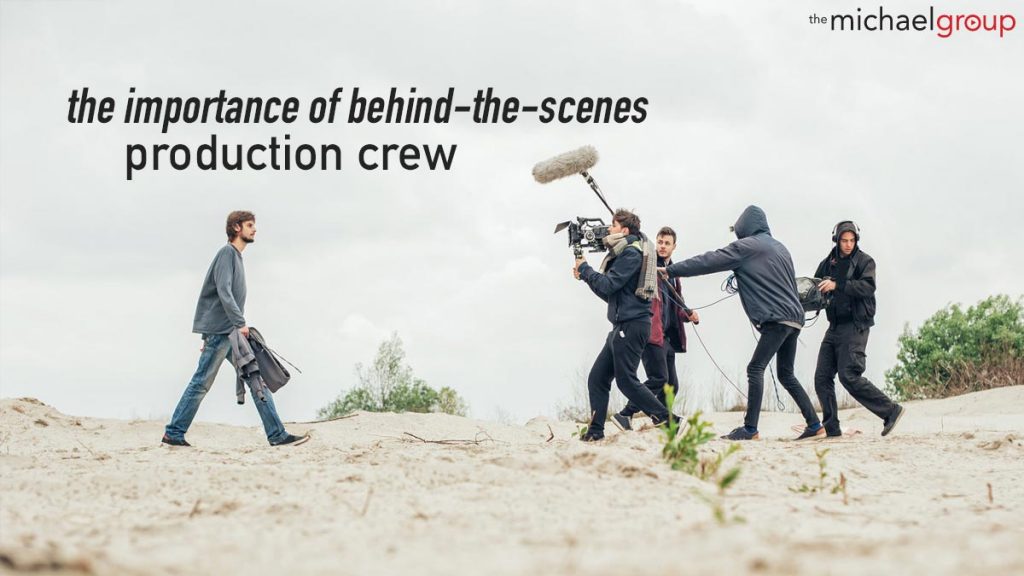The photograph captures an active behind-the-scenes moment on a film set located on a beach with light brown sand dotted with sparse, green vegetation. At the top left of the image, black text reads "The importance of behind-the-scenes production crew," highlighting the essential role of the crew in film production. On the top right, "The Michael Group" is prominently displayed, with "Michael" in black lettering and "Group" in red.

In the center of the photo, an actor is walking across the sandy terrain toward the camera crew. He sports a long-sleeve gray shirt, blue jeans, and sneakers, holding a gray jacket in his right hand. The actor has brunette hair and a beard.

To the right side of the image, the production crew is captured in action. The team consists of four men, all dressed in dark clothing. One crew member in a scarf, black sweatshirt, pants, and sneakers handles the camera. Another member, clad in a red jacket, holds a large gray microphone on a boom. Two additional crew members manage the wiring to prevent entanglement; one is dressed in a gray hoodie and black jeans, while the other wears black pants and a black coat.

This detailed depiction underscores the collaborative efforts of the production crew working seamlessly to film the actor as he walks along the beach.